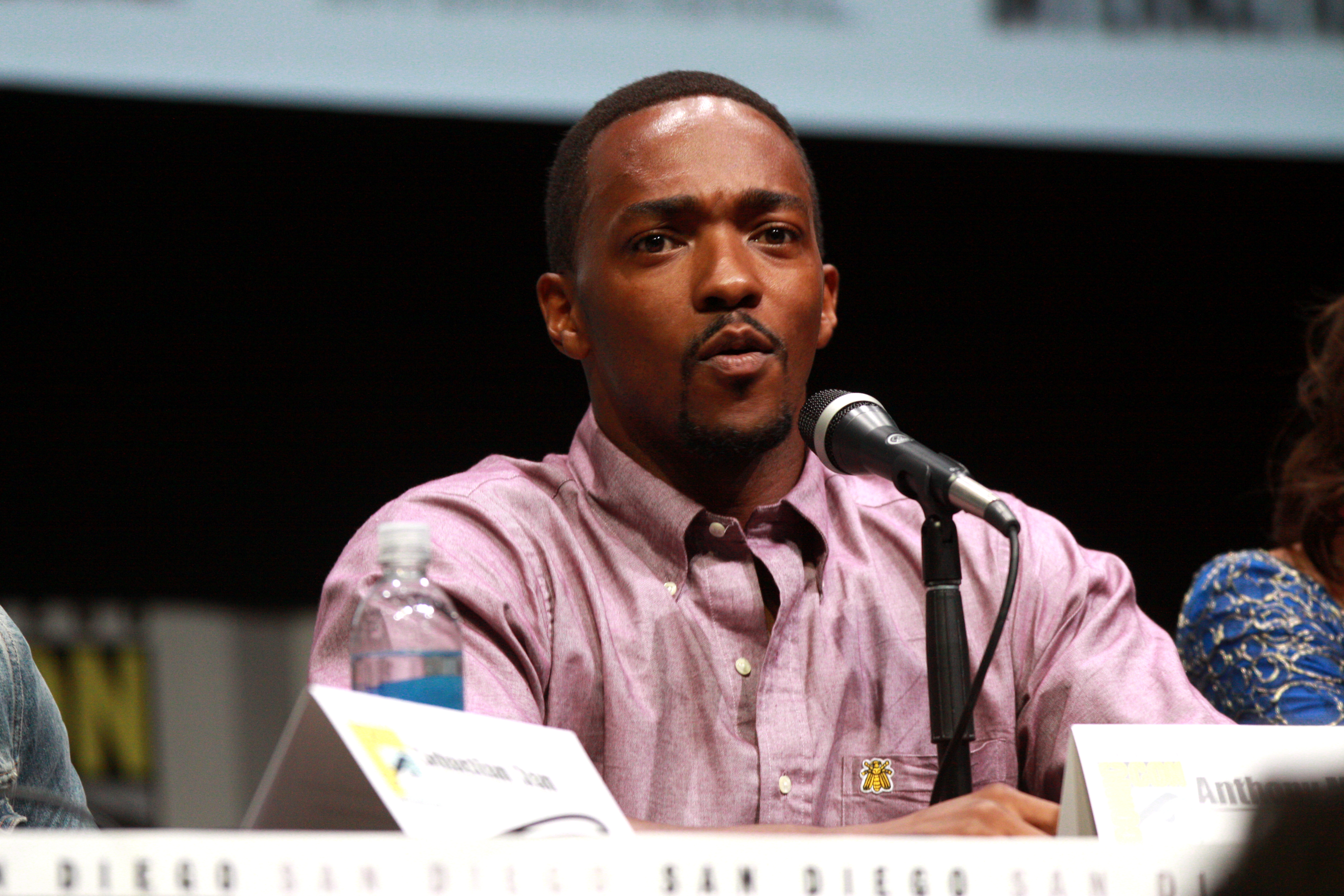A young black man, with short hair and a well-groomed goatee, sits at a table and appears ready to speak into a microphone positioned in front of him. He is dressed in a light purple, almost pink, button-down long-sleeve shirt, which features white buttons and a small logo of a yellow bumblebee. On the table, in front of his right shoulder, there is a clear water bottle and several folded name placards, one of which partially displays the letters "A" and "T." The background is predominantly black with a hint of white at the top, and next to the man on his left (camera right), a woman with medium brunette hair and a blue top adorned with a lacy gold-colored pattern is partially visible. The bottom part of the image features text that reads "San Diego" multiple times.